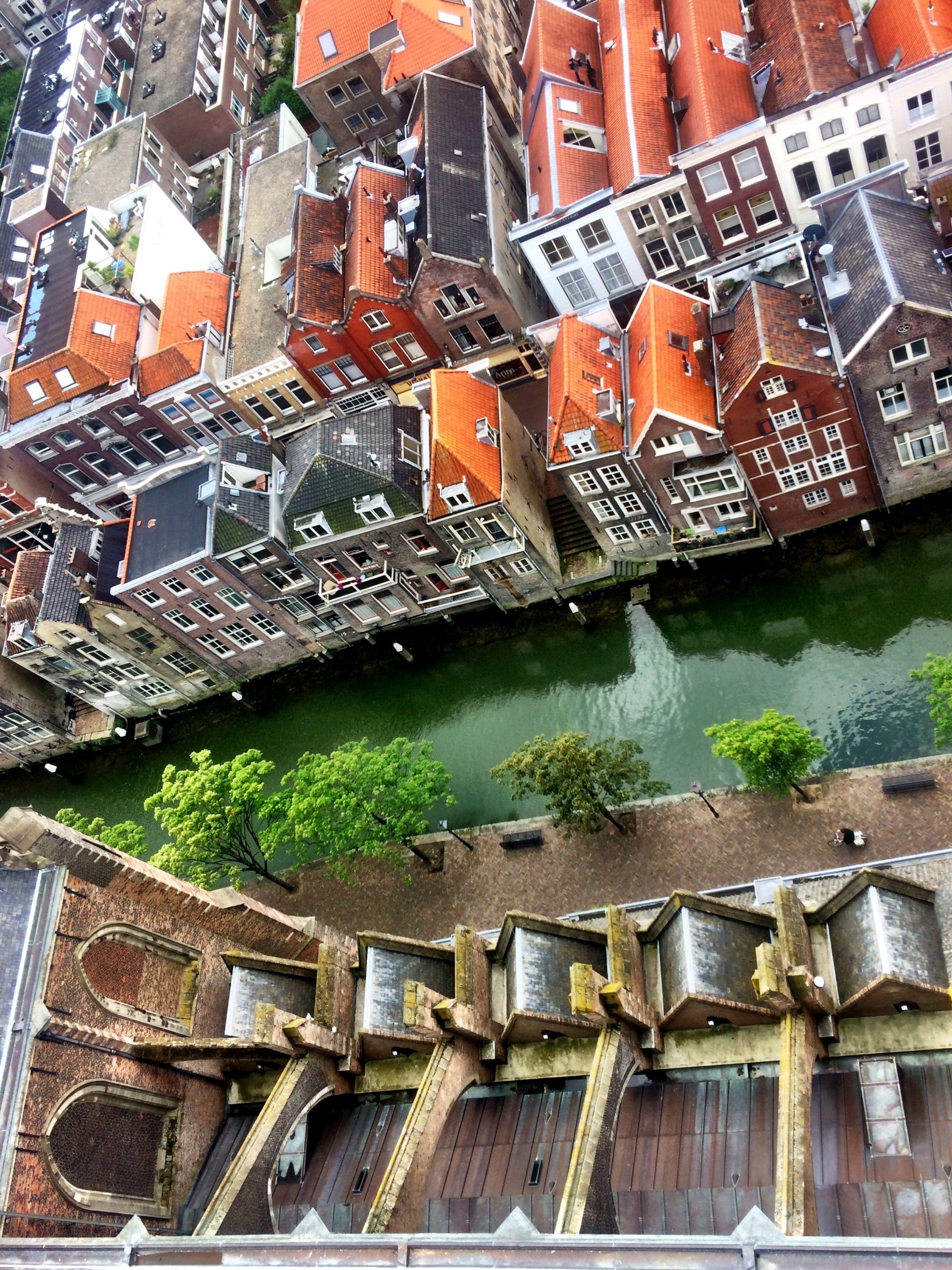This is an aerial view of a European town, possibly resembling Amsterdam, featuring a network of densely packed homes and buildings. The photograph, taken from a high altitude, showcases a rich variety of architectural styles and vibrant roof colors, ranging from orange, red, and burgundy to gray, brown, and white. The homes, many of which are tall, up to three stories or more, are tightly arranged front to back and side by side along the banks of a narrow, dark green waterway that runs straight down the middle of the image. Alongside the waterway, lined with trees, there is a walkway with benches. Toward the bottom and sides of the canal, smaller, older homes with brown roofs can be seen. Meanwhile, some of the larger buildings, possibly including a church with cathedral-style windows and tall peaks, dominate the landscape with their distinctive architectural features. The rooftops, mostly V-shaped but with a few flat-roofed structures, add a dynamic texture to the scene, making it a picturesque depiction of a charming European town from above.